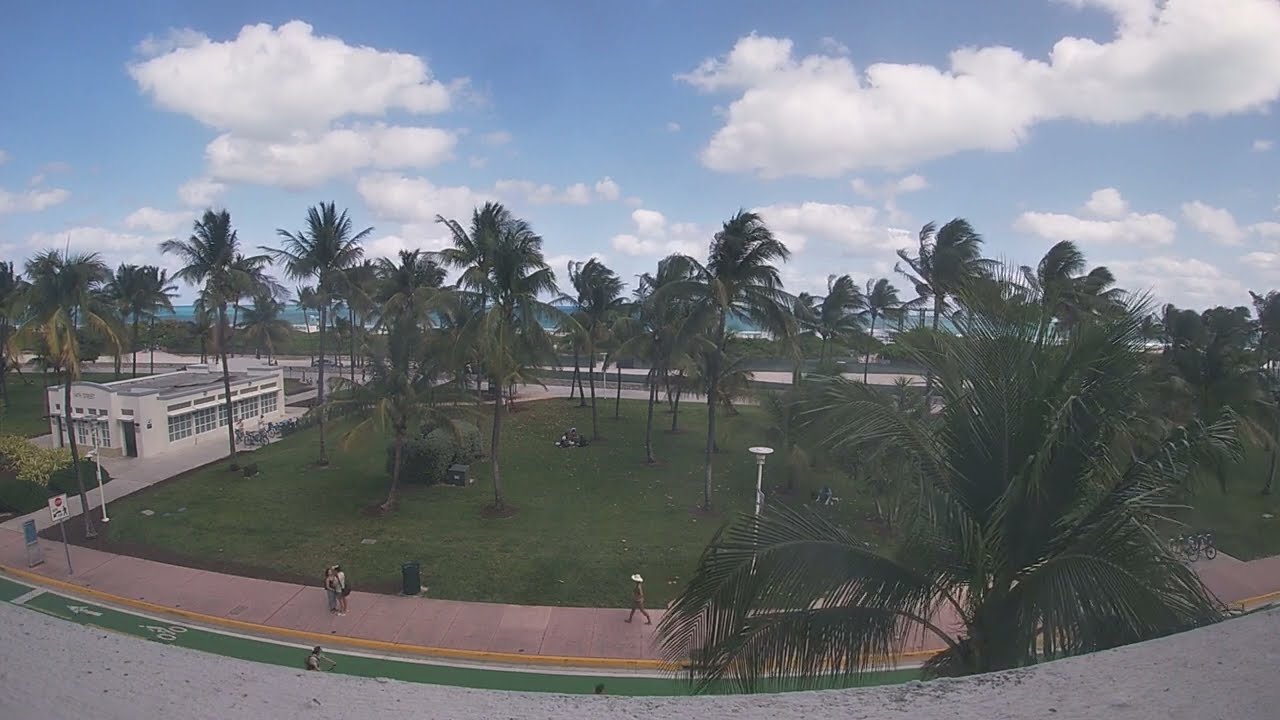The photograph, taken from a high vantage point, possibly a balcony or a concrete platform, showcases a wide-angle view of a park area with a distinctive fishbowl effect. At the bottom of the image, a gray concrete border or ledge is visible, hinting at the photographer's elevated position. Below, a sidewalk weaves through a grove of palm trees, where people can be seen walking. Adjacent to the sidewalk is a green bicycle path, which features one bicyclist.

To the left, a long, narrow white building with numerous glass windows stands prominently, possibly a store or a campus facility, suggesting a university-like setting. The area is populated with several people sitting on the grass, surrounded by the lush greenery of palm trees. In the far background, beneath a partly cloudy sky with thick, fluffy clouds, a glimpse of bluish-green ocean hints at the proximity to a beach. The entire scene is bathed in natural daylight, giving it a lively, outdoor ambiance.